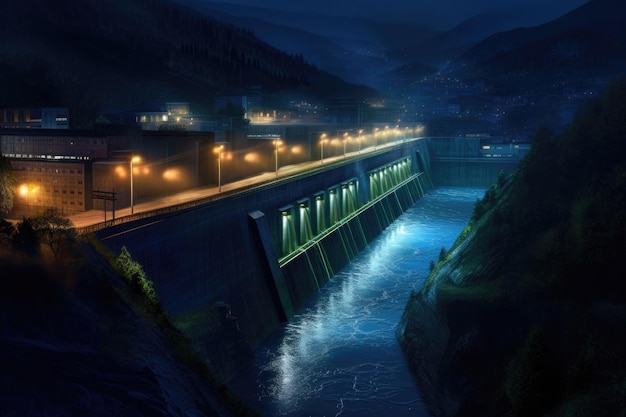The image is a nighttime, AI-stylized photograph of a dam with water forcefully flowing through various parts, creating white, choppy waves below. The dam structure, illuminated by streetlights, hosts a road on top with evenly spaced lights casting a warm glow over the scene. Adjacent to the dam, a stream runs parallel, reflecting the light. The area surrounding the dam includes boxy brown buildings to the left, a hint of architectural regularity against the natural backdrop. The right side of the dam transitions into a green mountain, adding to the dramatic scenery. The background is dominated by towering dark blue mountains shrouded in a foggy ambiance, interspersed with distant lights from buildings that dot the landscape far beyond the immediate horizon.